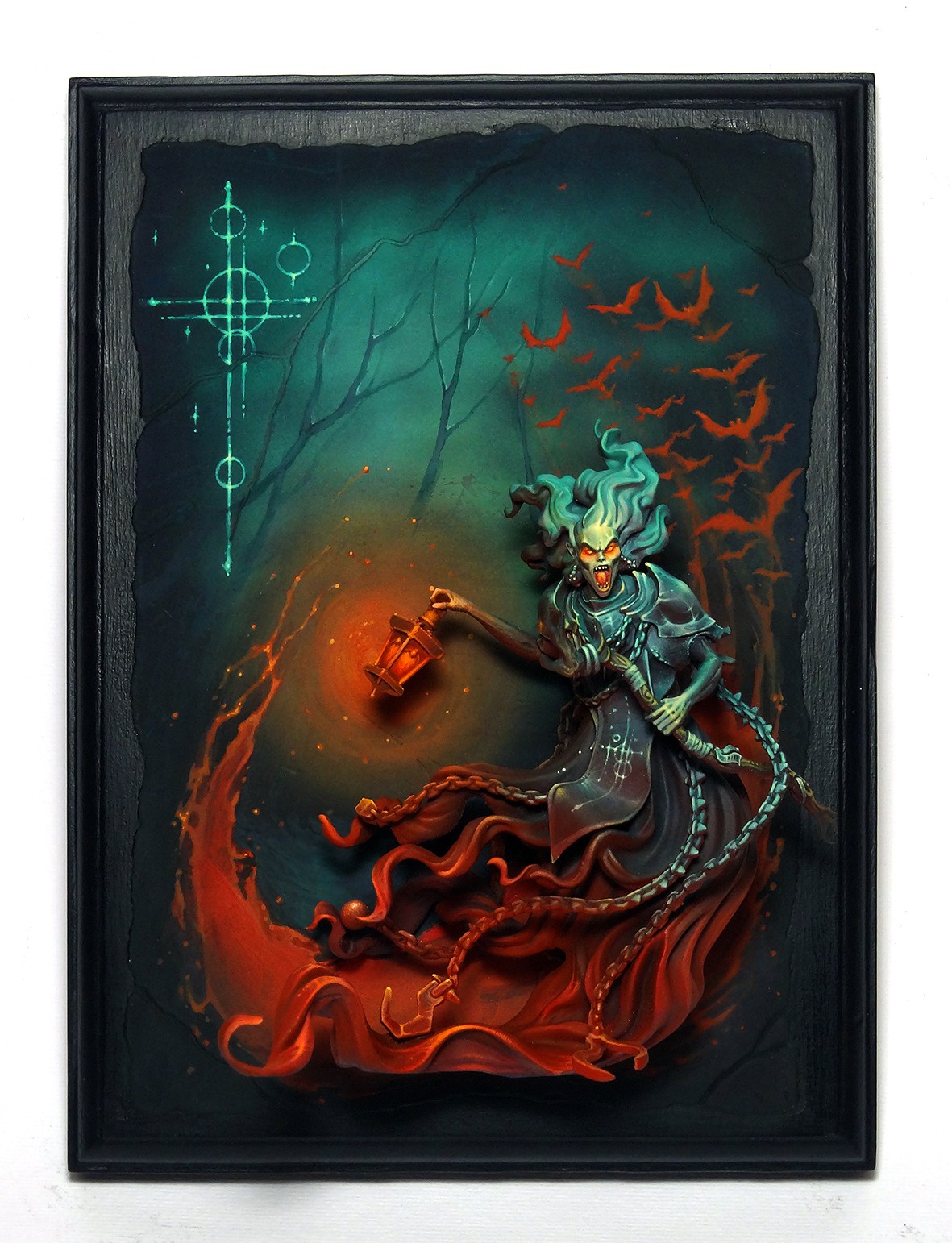In this striking digital illustration, a fearsome demon or bog witch emerges menacingly from a dark, leafless forest. The eerie scene is dominated by her imposing figure, clad in a garment that transitions from dark blue at the top to a sinister blood-red tide at the bottom. Chains and metal adorn her sinister form, complemented by armor around her shoulders and neck. Her glowing red eyes and wide-open mouth add to her terrifying presence, while long, flowing hair trails behind her. In her right hand, she clutches a red lantern, illuminating the dark scene. Reddish bats swarm around her, enhancing the dreadful atmosphere. To her left, a glowing neon green rune or symbol adds a mystical touch. The background features a few barren trees, contributing to the overall dark and haunting mood. The artwork, rich in red, teal, and dark tones, appears to be a digital creation, possibly intended for print and framing in a tall, rectangular format.